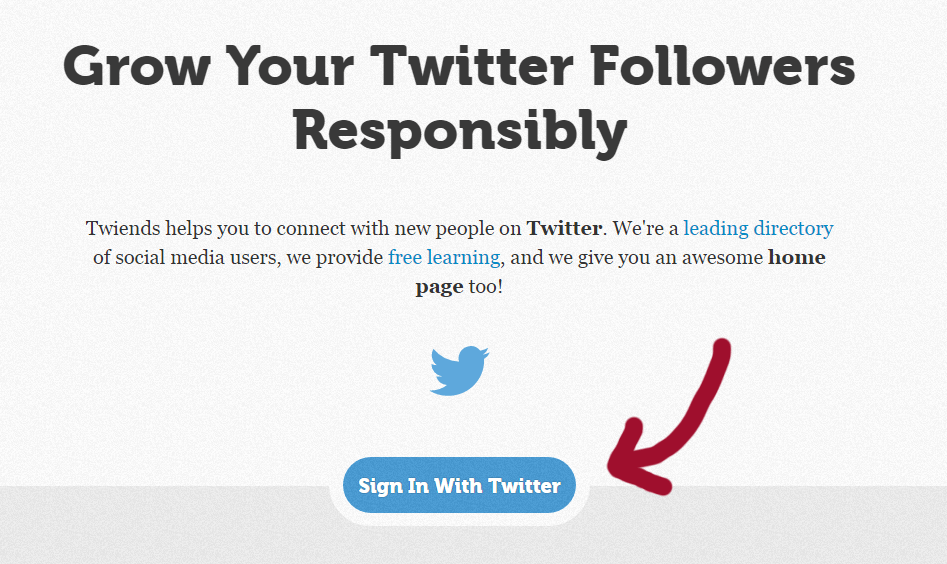Here is a polished and detailed caption for the image:

---

The image is a screenshot of a webpage with the headline "Grow Your Twitter Followers Responsibly" in large, bold black text against a light gray background. Beneath this, in small black text, it reads: "Twins helps you connect with new people on Twitter," with "Twitter" highlighted in bold. The next line states, "We're a leading directory of social media users," with the phrase "leading directory" in blue. Following this, the text says, "We provide free learning," with "free learning" in blue, and continues with, "and we give you an awesome home page!!" where "awesome" is in bold.

Below this text is the Twitter logo: a blue bird facing to the right, with extended wings and a circular body, depicted as a cartoon silhouette. Underneath the logo, there is a blue rectangle with rounded edges featuring the white text "Sign in with Twitter." At the bottom of the screenshot, a dark red, hand-drawn arrow points to the "Sign in with Twitter" button. This arrow is notably thick, matching the thickness of the "Grow Your Twitter Followers Responsibly" text. The font style for "Grow Your Twitter Followers Responsibly" and "Sign in with Twitter" is the same, while the rest of the text is in a thinner, simpler font. A gray line marks the bottom boundary of the screenshot.